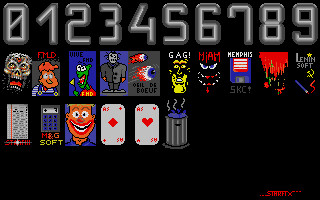The image features a small digital screen displaying what appears to be a game interface or a menu for games. The backdrop is a solid black, with the numbers 0 through 9 displayed prominently in white across the top. Just below these numbers is a row of ten portrait-oriented rectangles resembling the backs of playing cards, colored in various shades of red, blue, black, and gray. These rectangles showcase cartoony yet somewhat sinister-looking characters.

In the subsequent row beneath those, there are five additional cards. The first three appear face down, while the remaining two are face up, revealing the Ace of Diamonds and the Ace of Hearts. Adjacent to these cards is a rectangle resembling a calculator, differing in appearance but matching in size. Finally, in the bottom right corner of the screen, there is some small, unreadable text written in red.